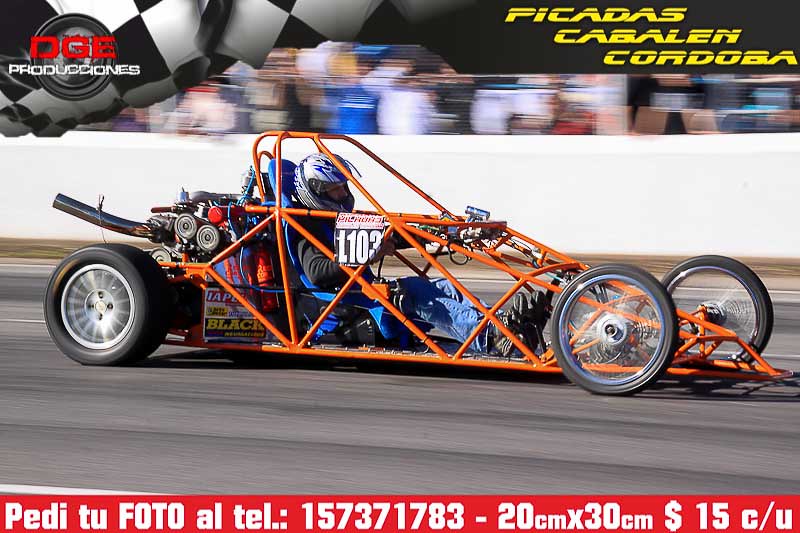This horizontal rectangular poster features a full-color photograph taken outdoors during a daytime car race. The main focus is a skeletal race car with no body, sporting an open metal frame and four visible wheels. At the rear of the car is a motor with an exhaust pipe extending outward. The driver is prominently seated with his back to the motor, legs stretched out along the bottom of the frame, clad in a blue racing suit and a crash helmet with a visor. The car appears to be moving at high speed, evident from the blurred stands packed with spectators behind a white wall. Enhancing the racing atmosphere, the upper left-hand corner of the image showcases a superimposed checkered flag and the logo "DGE Producciones," while the upper right-hand corner features golden Spanish text: "Picadas, Caballon, and Cordoba." A red banner runs along the bottom of the poster displaying white text, including details such as a phone number, the print size, and pricing information. The dynamic composition and vibrant elements make this piece a compelling advertisement for the thrilling race.